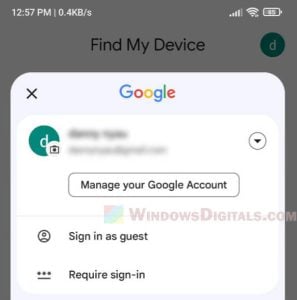**Caption:**

This image is a smartphone screenshot partially capturing a web page at 12:57 PM. The status bar at the top displays a battery icon at approximately 85% and a Wi-Fi connection indicator. The background features a gray dim overlay with the text "Find My Device" prominently displayed. In the center, there is a green circle containing a white "D."

The upper portion of the screen shows the Google search bar with the Google logo, followed by a green circle containing the "D" again, adjacent to a camera icon. Below this, the text "Manage your Google Account" is visible with a drop-down arrow to its right.

A watermark at the bottom reads "windowsdigitals.com" accompanied by a logo consisting of a square divided diagonally into green, blue, and yellow sections from the top left to the bottom right. Additionally, there is a "Sign in as Guest" option near a user icon, next to three dots underlined with the text "Require Sign-In."